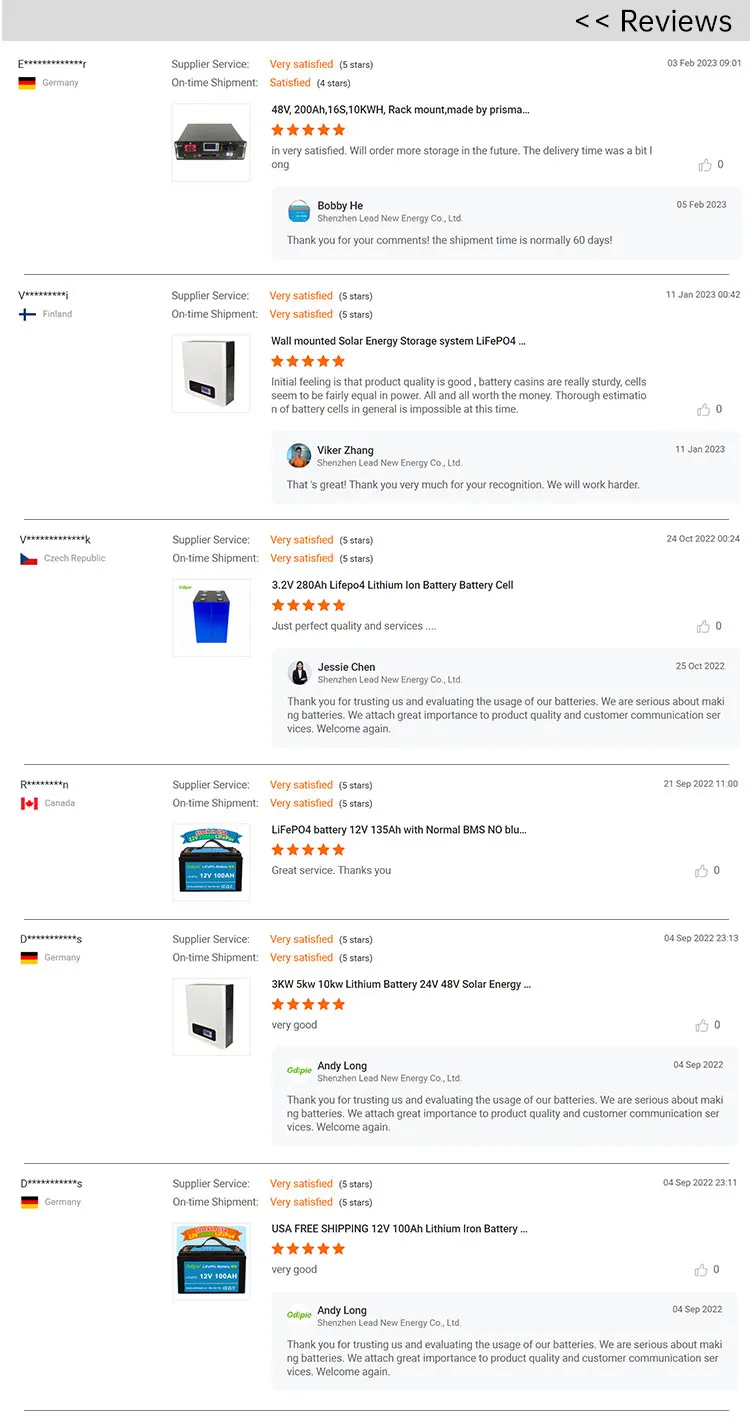This image showcases a neatly organized list of five-star reviews for six different products, each represented alongside flag icons indicating the country of origin. The reviewed products are displayed in a row, beginning with what appears to be a radio, followed by a processor, and then several battery-related items. Each product description includes the date of the review, though details about the reviewer or the business providing the products are not specified. All the five-star ratings are uniformly colored in a bright orange hue, emphasizing the highly positive feedback received for each item.